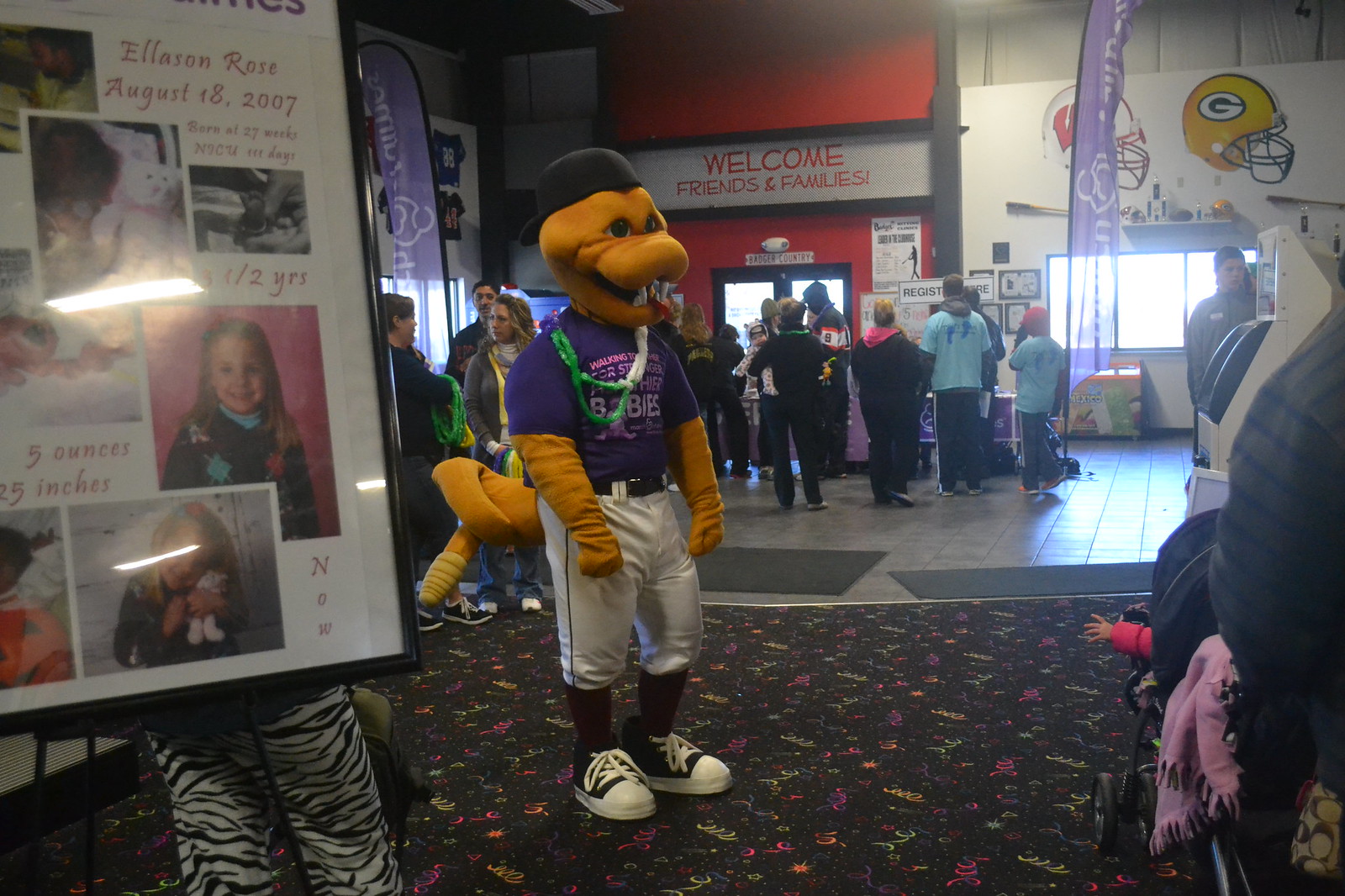In an indoor venue, a mascot dressed in an elaborate costume stands prominently at the center of the image. The mascot resembles a large rattlesnake, complete with a long tail that ends in a distinct rattle. It wears a russet-colored headpiece with a black baseball cap worn backward, and its snake head features fangs and a protruding tongue. The costume includes a purple short-sleeved shirt, black and white sneakers, and brown gloves sticking out from the arms. The figure's shorts, resembling black and white athletic wear, only partially cover its legs, which are adorned with black socks.

The backdrop reveals a bustling environment with men, women, and children milling around. The carpet underfoot is multicolored, adding vibrance to the setting. Behind the mascot, there is an entrance flanked by a red wall and topped with a sign that reads, "Welcome Friends and Families" in bold, red letters.

Further back, the wall features a large window emitting a soft, diffused light and a sign adorned with football helmets, including one identifiable as the yellow helmet with the white “G” logo of the Green Bay Packers. To the left of the mascot, set against the backdrop, there is a framed photograph display on the ground. The sign commemorates "Ellison Rose," detailing birth information and surrounded by images of the little girl. The detailed indoor decor, the mascot's intricate costume, and the surrounding people contribute to a lively and welcoming atmosphere.